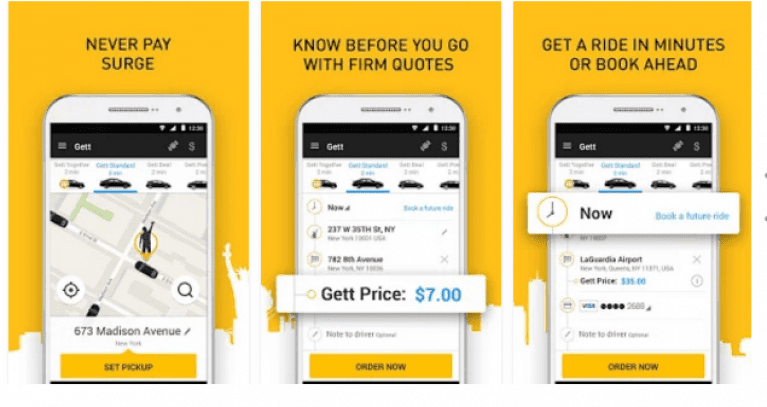This image features a triptych of promotional graphics for a mobile app, possibly related to transportation or ride-sharing services. Each graphic is set against a uniform yellow background, highlighting a simplified white cityscape in the backdrop and showcasing a different smartphone screen with app interface details. 

1. **First Image**: The caption reads, "Never Pay Surge." The smartphone appears to be a white iPhone with rounded edges. At the top of the screen, the status bar features the words "GET" on a black banner, flanked by a three-line icon on the left and two other icons on the right. The uppermost section displays typical status indicators: WiFi, network signal, battery charge, and current time. Below the "GET" banner, there are small car icons on a visible GPS map interface, indicating potential ride locations. At the bottom of the screen, a yellow button is prominently labeled "Set Pickup."

2. **Second Image**: The headline states, "Know Before You Go." Maintaining the same design aesthetics, this screen shows destination points and progress indicators in the form of circles aligned vertically. There is an overlay on the image showing the text "Get Price $7" along with a yellow button at the screen's bottom labeled "Order Now."

3. **Third Image**: The phrase "Get a Ride in Minutes, Book Ahead" tops this graphic. Similar in layout to the previous images, this screen features an overlay with the word "Now" and an illustrated clock symbol, suggesting immediate availability. The right side of the screen displays additional information, aligned with an interface indicating options comparable to previous images.

The cohesive design across all three graphics emphasizes ease of use and quick access, likely aimed at enhancing user experience for ride bookings.